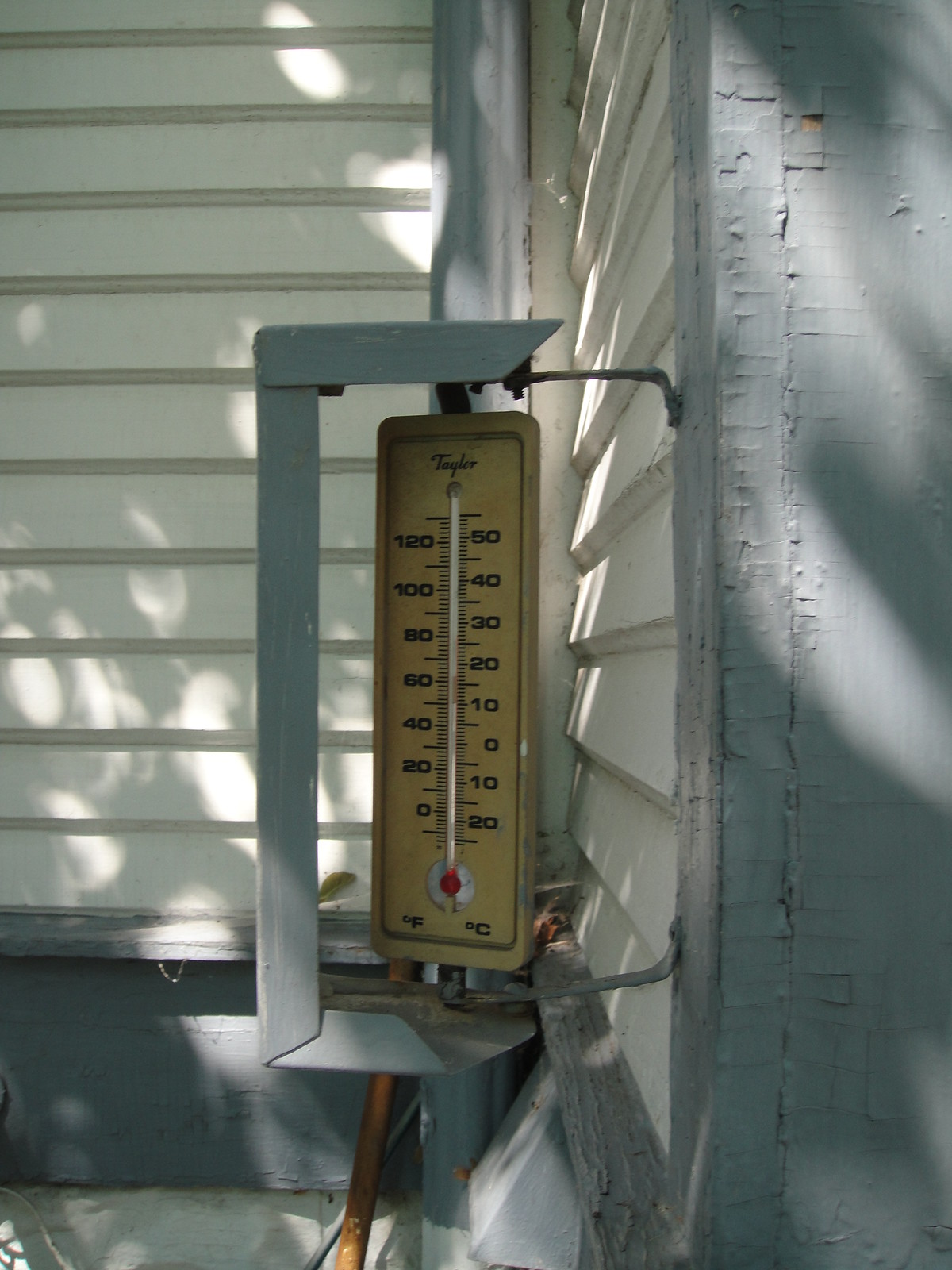The photograph, taken during the day, showcases a tan-colored thermometer with black numerical markings and the letters 'F' and 'C' indicating Fahrenheit and Celsius respectively. The thermometer, branded "Taylor" at the top in black font, features a red line running down its center. It is mounted on a metal pole affixed to a building with white siding, accented by gray detailing with peeling paint. Sunlight illuminates the siding, creating reflections on the gray paint and casting tree shadows. The building's architecture includes wood trim around the edges, and a small area of white concrete is visible at its base.